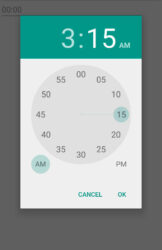The image is a vertically rectangular, blurry screen capture from a cell phone, featuring a gray background and a smaller pop-up window displaying a clock or alarm setting interface. At the top of the pop-up window, there is a green, horizontally rectangular banner with the time "3:15 AM" displayed on it. The digit '3' appears in a pale color while '15' stands out in bright white. This corresponds with the clock below, where the number '15' is highlighted by a light green circle. 

Below the main clock face, there are two smaller circles: the left one labeled "AM" and circled in light green, and the right one labeled "PM". At the bottom right corner of the pop-up window, there are two options, "Cancel" and "OK," both presented in green text. The overall setting suggests an interface where a user is likely adjusting or setting an alarm for 3:15 AM.